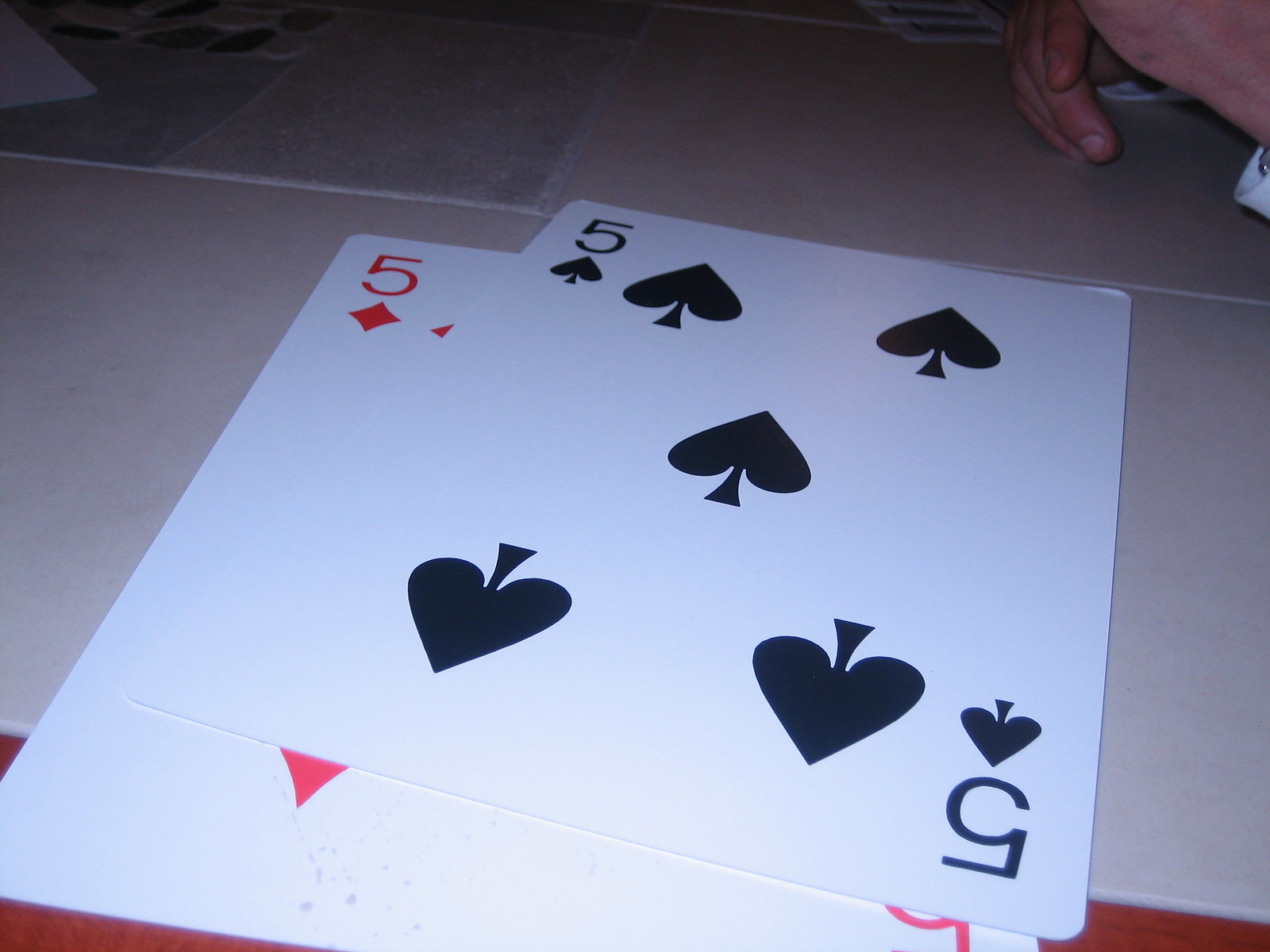In the image, two oversized playing cards rest atop a square-tiled table. The bottom card is a red five of diamonds, while the top card is a black five of spades. The close, low-angle perspective from which the photo is taken exaggerates the cards' size, making them appear to cover an entire tile on the table. In the upper right-hand corner, a hand dressed in a long white sleeve hovers slightly above the table, further emphasizing the cards' apparent largeness. The upper left-hand corner reveals a subtle change in the table's tile design, showcasing a mix of different rock patterns and shades of gray distinct from the rest of the table. Overall, the image plays with scale and perspective, creating an intriguing visual effect.